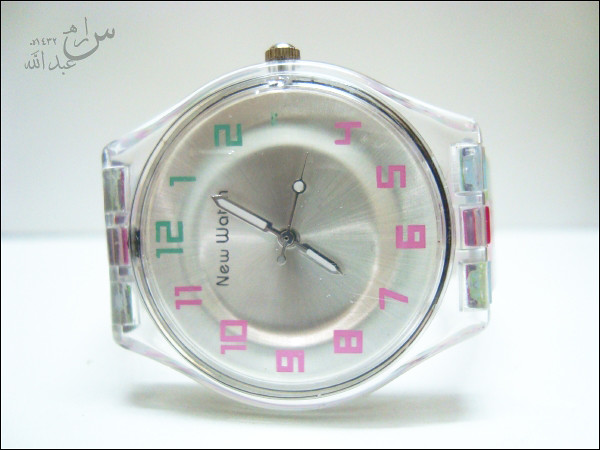This photograph captures a clear plastic wristwatch in an unconventional pose, lying on its side without any visible band or strap. The watch features a transparent casing accented with a combination of pink, green, and hints of a bluish tint. Its face, which has a silver or metallic background, prominently displays the brand "New Watch" at the top center. The numbering is unique, with 12, 1, and 2 in green, while 4 through 11 are in pink. The number 3 has been smudged off, leaving an empty spot. The time shown on the watch is 7:05, with the hour hand slightly past 7 and the minute hand pointing at 1. The hour and minute hands are silver with white inlays, and the second hand is silver with a circular white inlay. This close-up and detailed presentation hints at a possible advertisement for the watch brand.